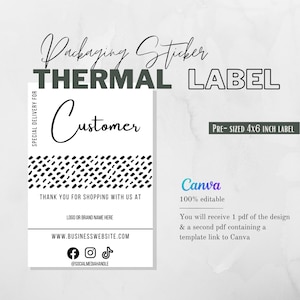This graphic advertisement for Canva features a detailed depiction of a packaging sticker thermal label. The ad showcases a pre-sized 4x6 inch white label designed for products being sold. The label’s main text is the word "customer" written in script at the top, followed by a diagonal black pattern resembling a tire tread. It includes a thank you message: "Thank you for shopping with us," as well as social media icons for Facebook, Instagram, and TikTok. Above the label, the text "Packaging Sticker Thermal Label" is displayed, with each word in a distinct font style. Canva's logo, in a gradient of blue and purple, appears prominently, noted as 100% editable. The design package promised in the ad includes one PDF of the label design and a second PDF containing a template link to Canva. The background of the ad features a periwinkle blue marbled square, adding an aesthetic appeal to the overall presentation.